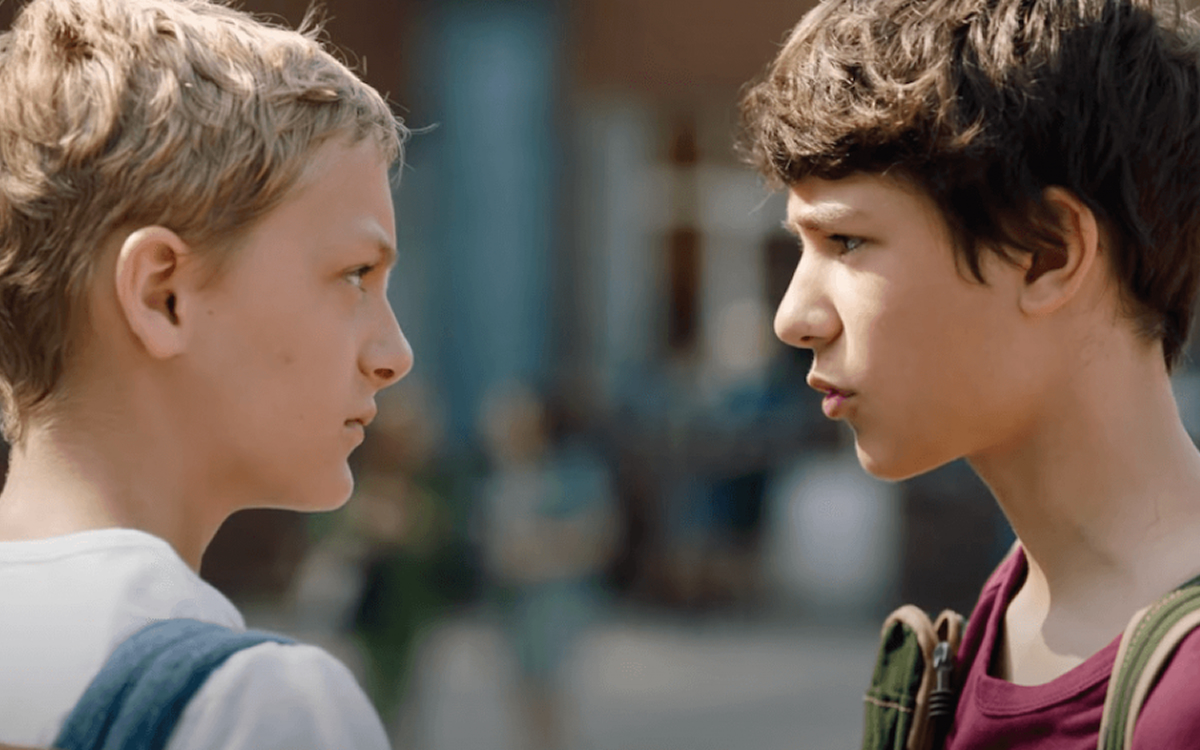In this image, two boys, approximately 8 to 12 years old, are captured in profile, intensely staring at each other with expressions that convey a mixture of concern, aggression, and concentration. The boy on the left, whose light brown hair contrasts with his white shirt, is seen with a blue backpack strap over his shoulder. His face, etched with anger, dominates the left side of the image. Opposite him, the boy on the right, with dark brown hair and wearing a dark red shirt with green backpack straps, appears equally agitated, as if about to say something. The background, a blurred blend of what could be a schoolyard or cityscape with indistinct figures, focuses the viewer’s attention on the palpable tension between the two boys.